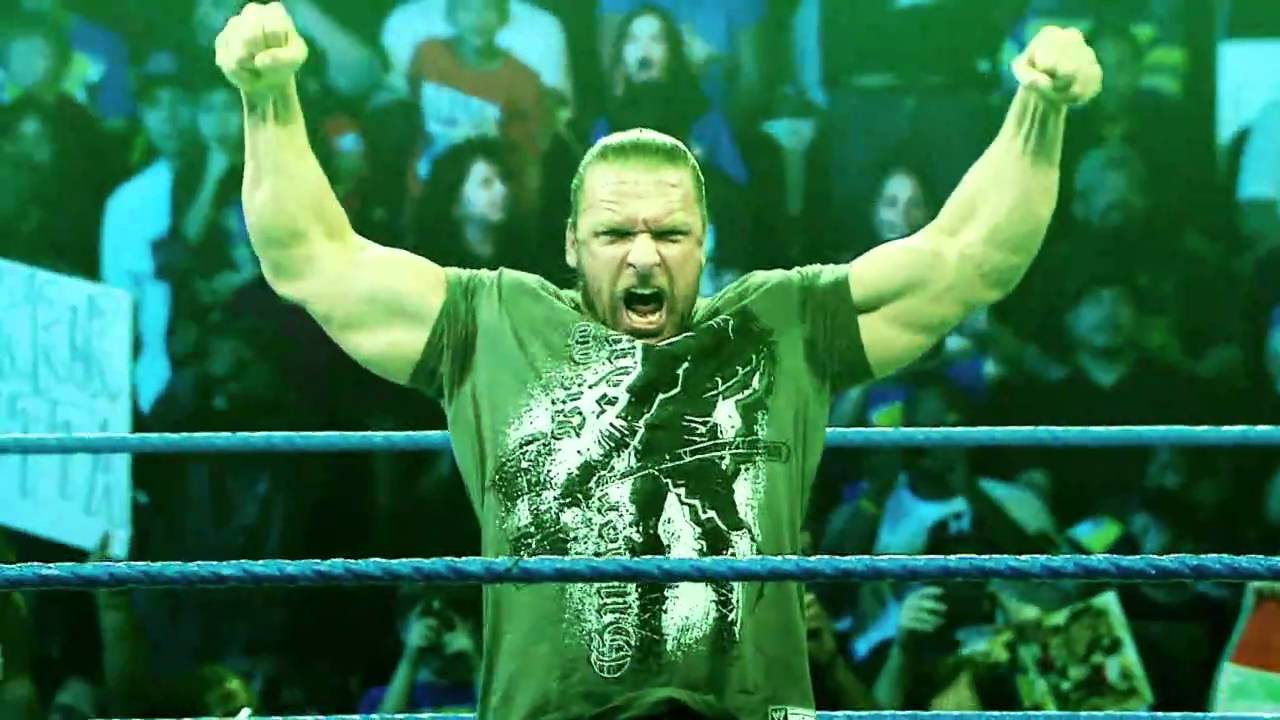The image captures a professional wrestler standing at the center of the ring, lifting his arms above his head and flexing his biceps. He has a ferocious expression on his face, mouth open as if shouting, conveying sheer intensity. The wrestler is wearing a green shirt adorned with a graphic of a man wielding a sledgehammer, which pops vividly against the scene. Sweat stains are visible under his arms, underscoring the physical exertion and heat of the moment. The ring ropes in front of and behind him are blue, framing his powerful stance. The crowd in the background is a blur of excitement, with some fans energetically holding signs and others capturing the moment with their cameras. One woman directly behind the wrestler has her mouth open, looking particularly thrilled, adding to the electric atmosphere. The green tint in the image suggests dynamic lighting within the wrestling arena, enhancing the dramatic effect. This poised and powerful image suggests the wrestler is either celebrating a triumphant victory or gearing up to showcase his dominance in the ring.